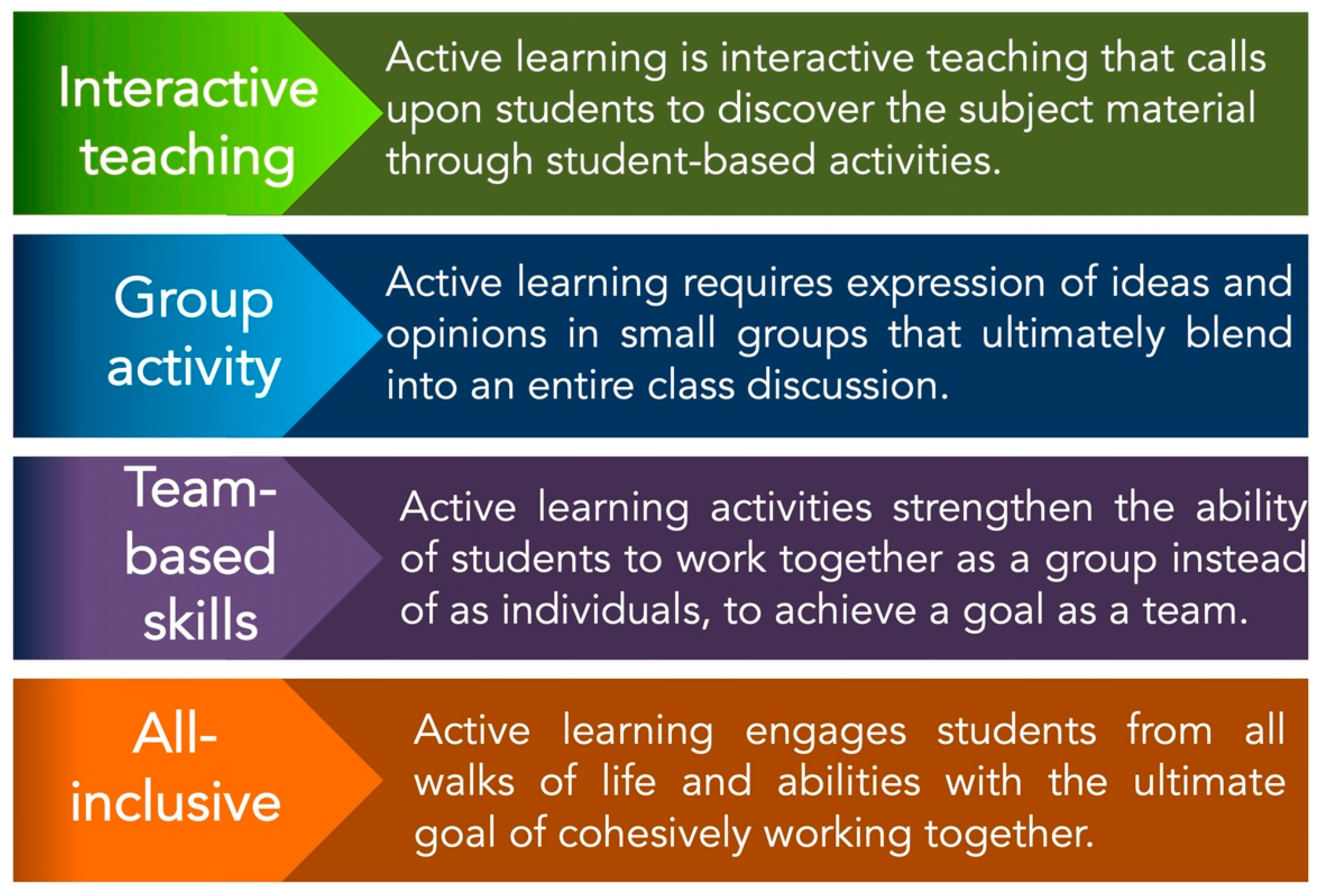The image consists of four color-coded panels, each illustrating different types of active learning and teaching methods. The top panel has a green background with white letters and is labeled "Interactive Teaching." It describes active learning as an interactive approach that encourages students to discover subject material through student-based activities. The second panel, with a blue background, details "Group Activity," highlighting that active learning necessitates the expression of ideas and opinions in small groups, which ultimately blend into a full class discussion. The third panel, in purple, is focused on "Team-Based Skills." It explains that active learning activities enhance students' abilities to work together as a team to achieve common goals. The bottom panel, in an orange background, is titled "All-Inclusive." It emphasizes that active learning engages students from diverse backgrounds and abilities, aiming for cohesive teamwork. Each panel uses a tapered design on the right side pointing to the detailed descriptions, with text color predominantly in white.